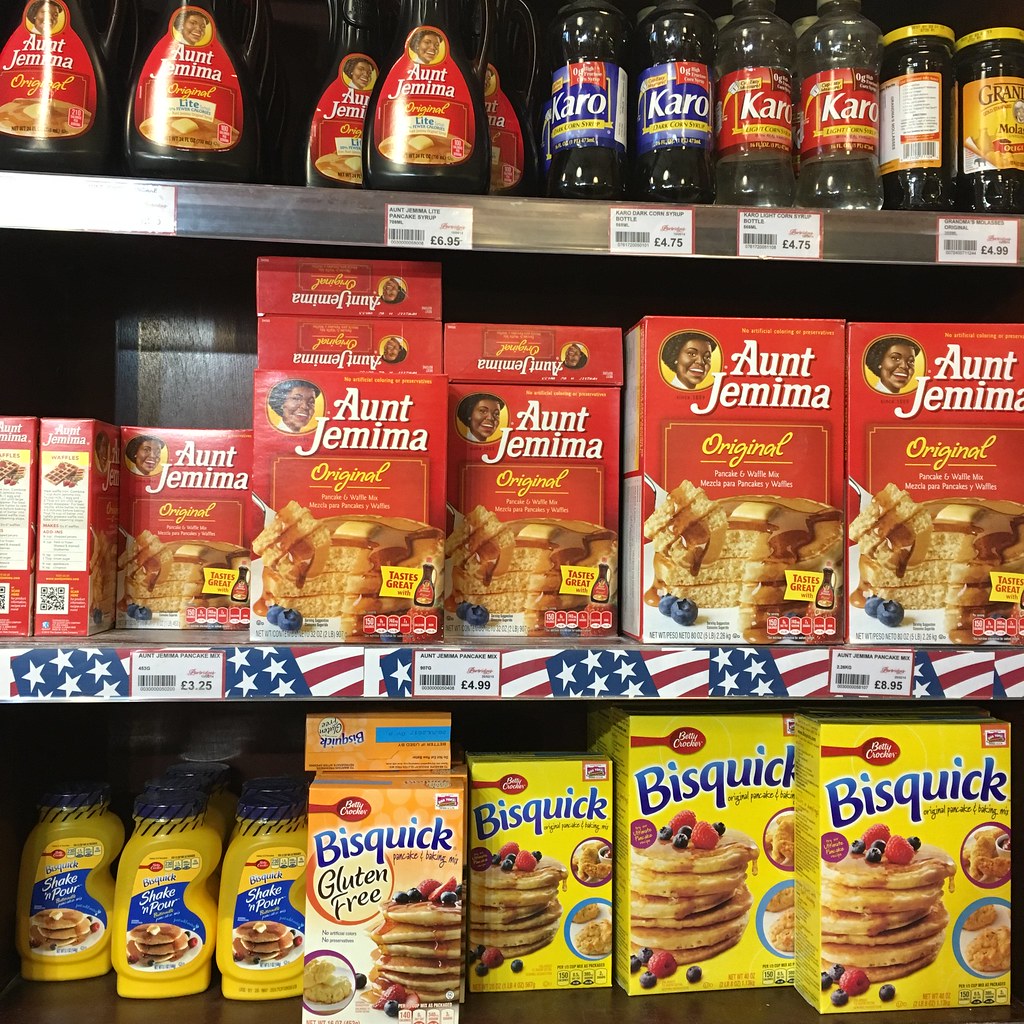The image showcases a well-organized grocery aisle dedicated to breakfast items. On the top shelf, there are five bottles of Aunt Jemima syrup priced at $6.95 each. Accompanying these are four bottles of Karo syrup—two with blue labels and two with red—each priced at $4.75. Additionally, a jar of molasses is positioned at the end of the top row, costing $4.99.

The second shelf features various sizes of Aunt Jemima pancake mixes. On the far left, there are small boxes of the original pancake mix priced at $3.25 each. In the middle, slightly larger boxes are available for $4.99, and towards the right, the largest boxes are priced at $5.95.

The bottom shelf is dedicated to Bisquick products. Starting from the left, it includes shake-and-pour Bisquick, a gluten-free Bisquick mix, small boxes, and large boxes of the regular Bisquick mix, each arranged in a neat row.